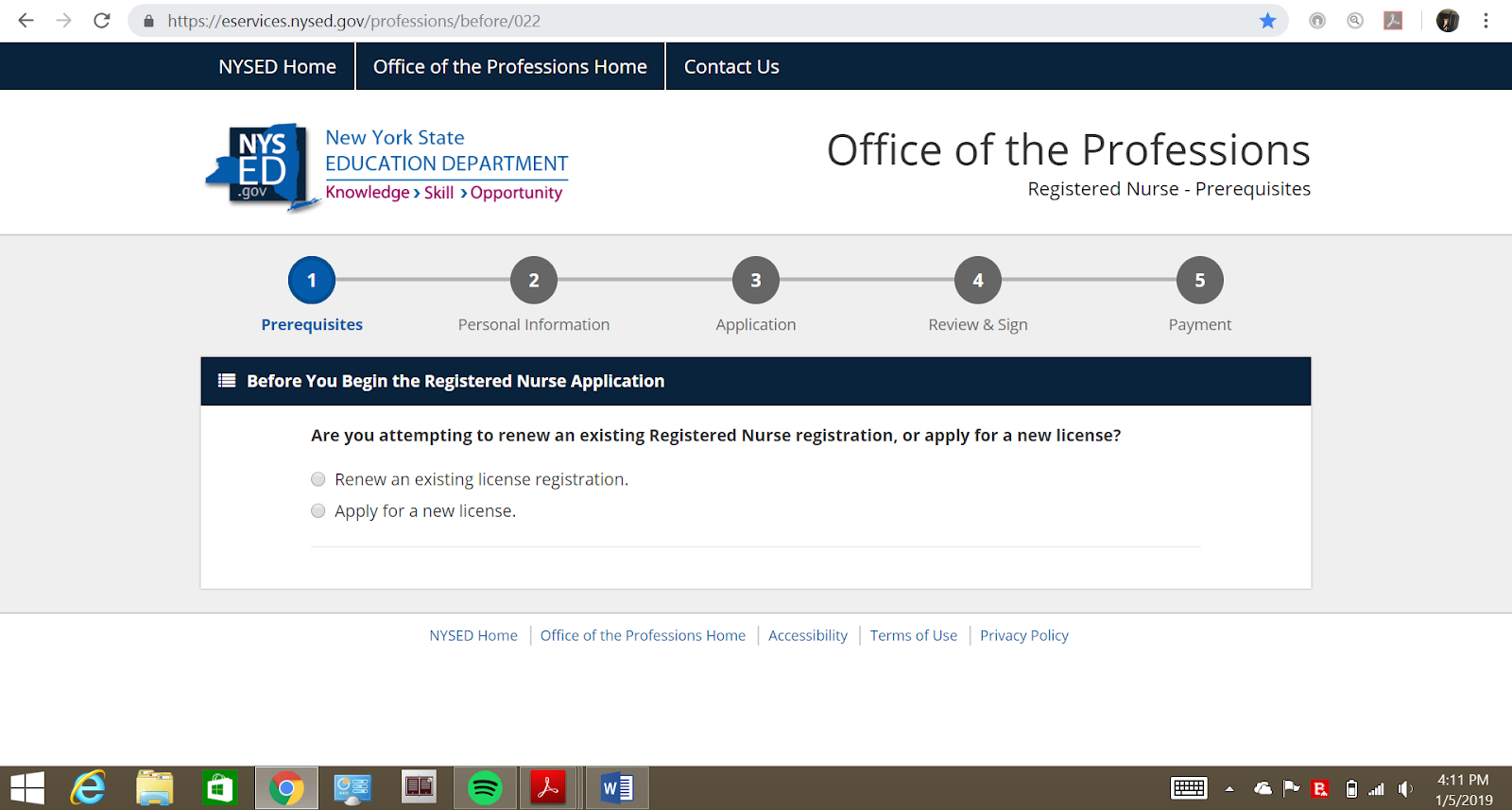Screenshot of the New York State Education Department's Website

The screenshot captures the New York State Education Department's (NYSED) official website interface. At the top, there is a blue navigation bar featuring links titled "NYSED Home," "Office of Professions Home," and "Contact Us," each separated by vertical dividers. Below the navigation bar, a blue-ribbon NYSED logo is prominently displayed, accompanied by the words "New York State Education Department." Underneath the department's name, the motto "Knowledge → Skill → Opportunity" is inscribed. 

To the right of the logo, the heading "Office of the Professions - Registered Nurse - Prerequisites" is displayed. Below this heading, a navigational chart outlines five steps in the application process: 1. Prerequisites, 2. Personal Information, 3. Application, 4. Review and Sign, and 5. Payment. 

A secondary blue bar below the chart reads "Before you begin the registered nurse application." Beneath this, the user is prompted with the question: "Are you attempting to renew an existing registered nurse registration or apply for a new license?" Two radio buttons are presented as options: "Renew an existing license registration" and "Apply for a new one," though neither is selected in the screenshot.

The bottom section of the page includes links for "NYSED Home," "Office of Professions Home," "Accessibility," "Terms of Use," and "Privacy Policy." The background of the entire webpage is white, creating a clean and professional appearance.